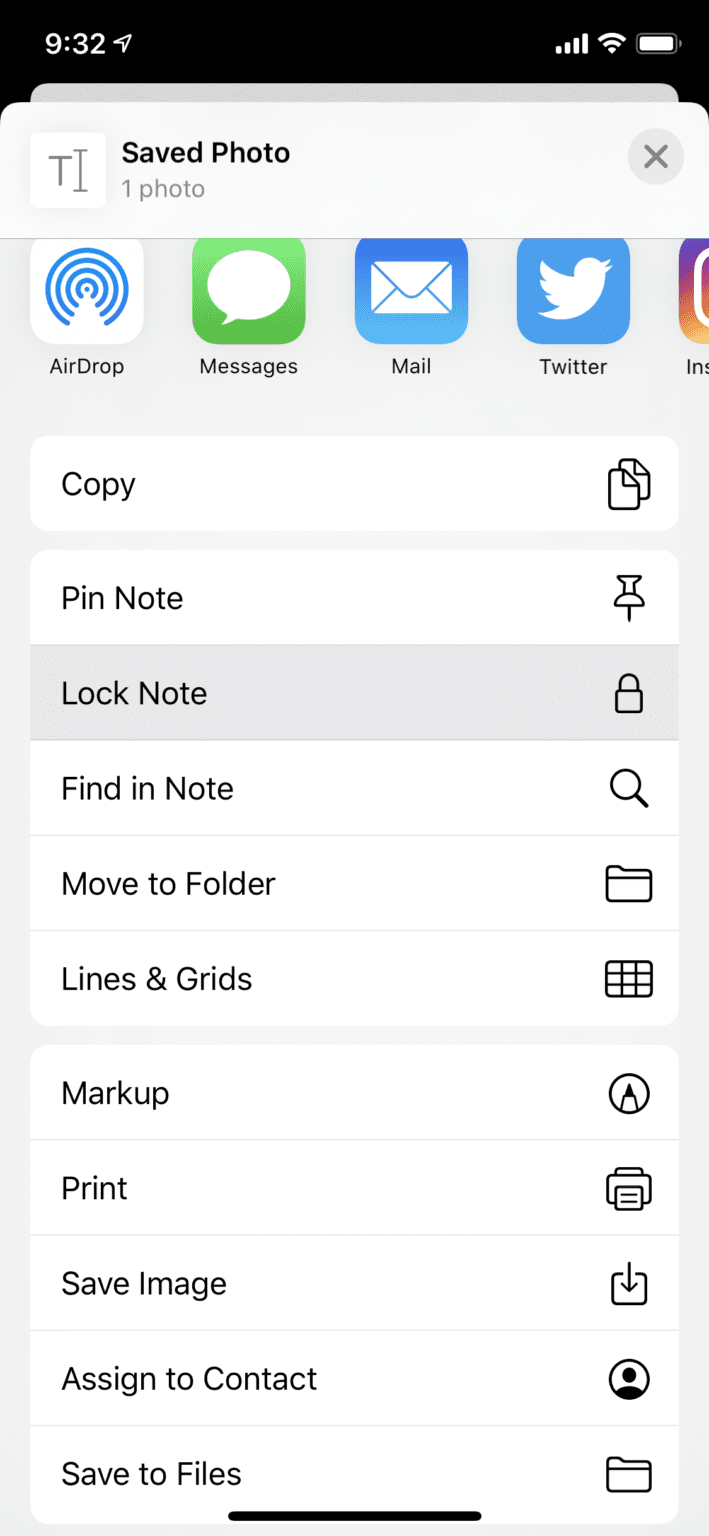This is a detailed screenshot of an iPhone interface, specifically displaying options for managing a saved photo. At the very top, the status bar is outlined in black, featuring the time "9:32" in white font on the left, and signal indicators on the right, including full cellular signal bars, a strong Wi-Fi signal icon, and a fully charged battery icon.

Below the status bar is a menu of share options for the photo. The visible options include "AirDrop", "Messages", "Mail", and "Twitter," with the edge of the "Instagram" icon just peeking into view. 

Underneath, a more extensive menu lists further actions that can be performed with the photo: "Copy", "Add to Notes", "Lock Note", "Find in Note", "Move to Folder", "Lines & Grids", "Markup", "Print", "Save Image", "Assign to Contact", and "Save to Files". Each function is accompanied by a small corresponding icon to its right, providing a visual cue to the user.

Overall, the image showcases the extensive sharing and editing capabilities available within the iPhone's operating system for managing photos.